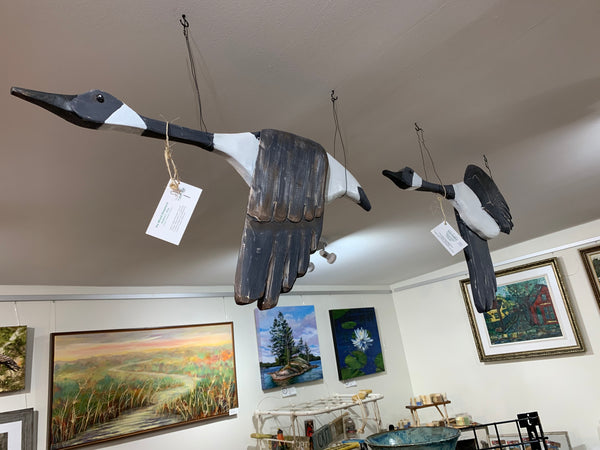This image depicts a detailed, realistic photograph of an interior exhibit space, likely a museum or art gallery. The walls, converging in a corner, are adorned with a multitude of framed artworks, including landscapes, nature scenes of trees and rivers, and depictions of houses and flowers. On the table below, partially cut-off items can be seen, suggesting the presence of additional displays or merchandise.

Suspended from the ceiling by thin black wires, two intricately carved wooden geese, painted in striking black and white, are depicted in mid-flight. Positioned in the foreground, the goose on the left, closest to the viewer, showcases a detailed pattern with a black head, a streak of white at the neck's beginning, followed by black through the neck, and a white body with black wings and tail. Its companion, further in the background, mirrors this design. Both geese have small tags attached to their necks with straw ties, indicating that these unique pieces are likely for sale. The overall scene captures a serene and evocative moment within this well-curated art space.